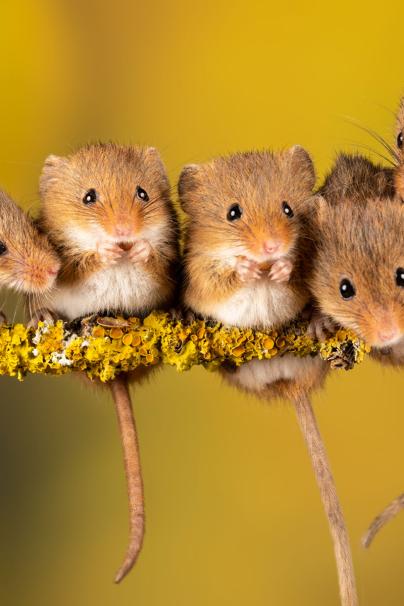The image features five adorable tan mice with white chests and underbellies, perched on yellowish-green flowers against a blurry yellow background. Two mice are fully visible in the center with their paws raised to their mouths, seemingly eating nuts. The third mouse is mostly in frame on the right, while the fourth mouse's face peeks in from the left. The face of the fifth mouse is just partially visible on the far right. Each mouse has small, round black eyes and pink noses, with varying tail colors—one tan and another more pinkish. The background darkens slightly towards the left, providing a subtle gradient that enhances the scene's warmth and charm.